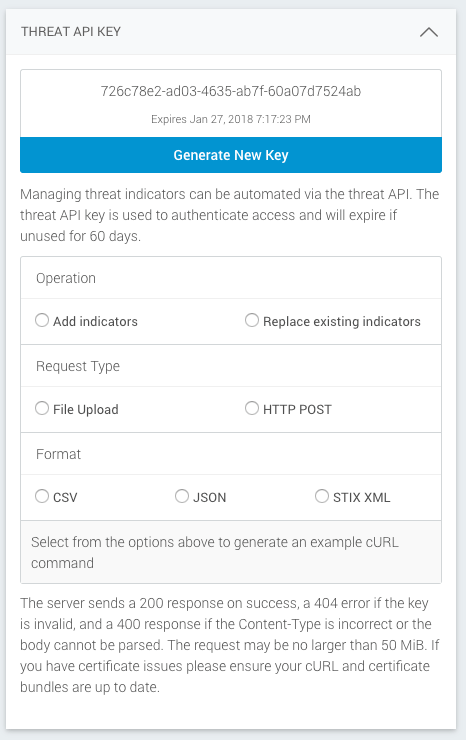This is a detailed screenshot from a phone screen displaying a software interface for managing threat indicators via an API. At the top of the screen, the text reads "Threat API Key," indicating that this part of the application is responsible for handling API key authentication. A light blue button labeled "Generate New Key" is prominently placed at the top, offering users the option to create a new API key.

The interface explains that the Threat API Key is critical for authenticating access and mentions that any unused key will expire within 50 to 60 days. Below this explanation, there are various radio buttons and selection options categorized under "Operation," which includes options to "Add Indicators" and "Replace Existing Indicators." Another category labeled "Request Type" offers choices like "File Upload" and "HTTP Post," with an additional section for selecting the format.

At the bottom of the screenshot, instructional text clarifies the server responses: a "200 response" indicates success, while a "404 error" denotes an invalid key. A "400 response" is returned if the content type is incorrect or if the body cannot be parsed.

The overall design of the application is minimalist, with a white background. The "Generate New Key" button stands out as it is light blue with white text, adding a touch of color to the otherwise monochromatic interface. The screenshot effectively captures the application's functionality for generating and managing API keys on a mobile device.